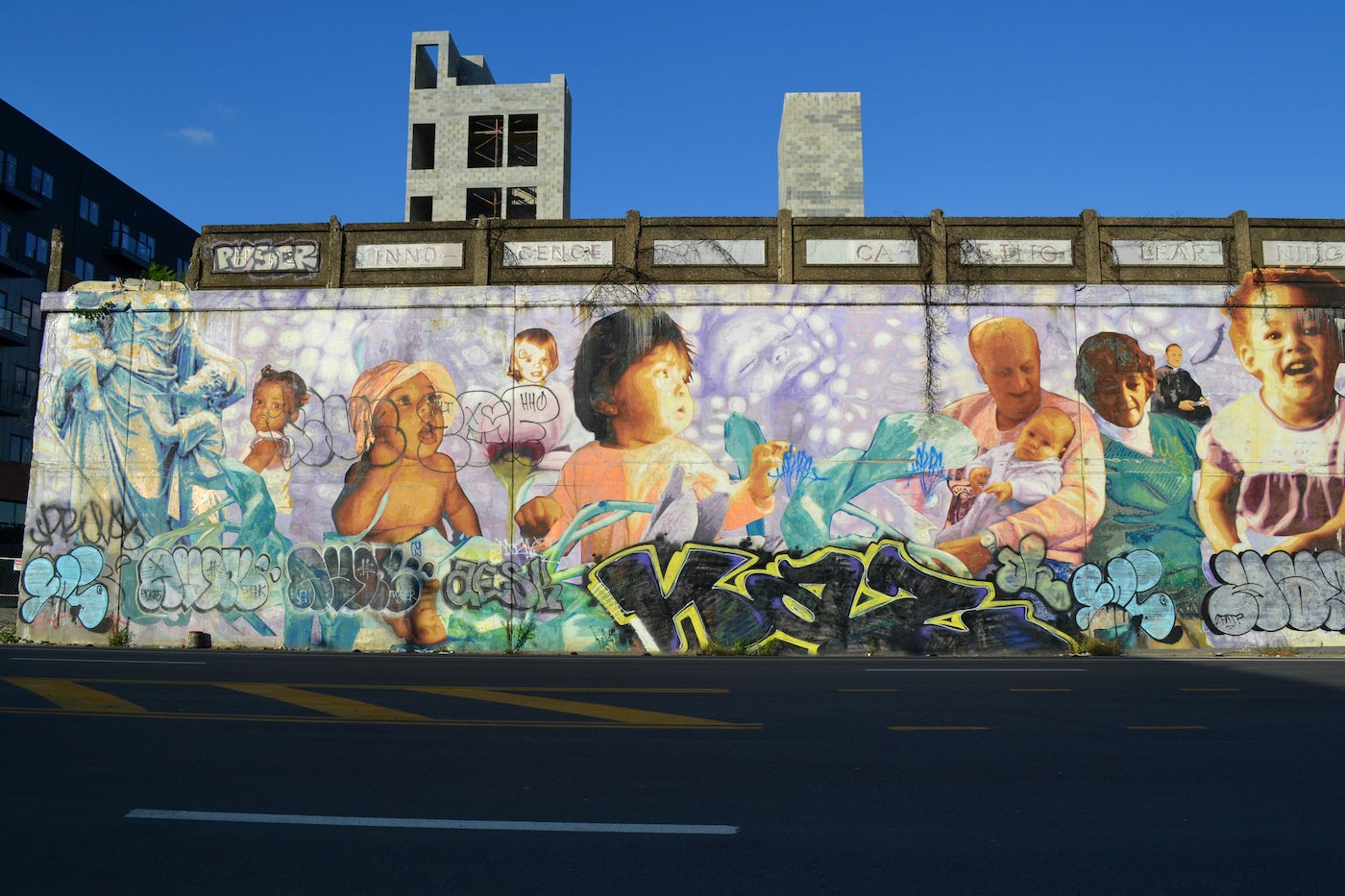This image captures a vibrant, yet heavily defaced, mural on the side of a building that stands about three or four stories tall. The mural features detailed and diverse depictions of babies, toddlers, adults, and grandparents, possibly serving as a memorial to these individuals. The central figures include a black baby on the left, another black baby to the right, an Asian baby, and a white baby. On the far right, a black baby is painted alongside a man dressed in a black priest robe. Prominently situated are two grandparents: a grandfather in a pink sweater cradling a baby, and a grandmother in a green sweater. Amidst these figures, there's an image of a statue with a small child clinging to it.

Despite its celebratory nature, the mural has been marred by graffiti, including gang signs scattered at the bottom. The mural's background is filled with a mixture of colors, predominantly purple, enhancing the images, yet overlaid by various tags and writings. The scene is set against a clear sky with daylight illuminating the building and the street in front, which features white and yellow-striped lines along a parking lot and street, completing this complex urban tableau. Towers rise into the sky behind the building, adding a contrasting modern element to the mural’s more personal and historical feel.